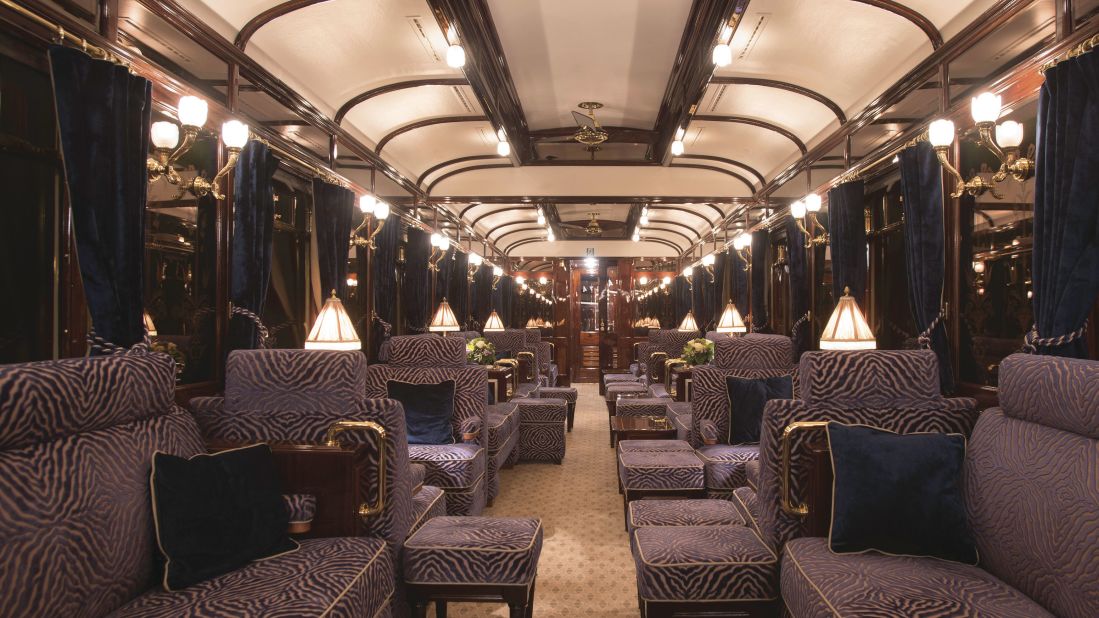This color photograph depicts the interior of an elegantly refurbished train car, reminiscent of an old-time passenger or Pullman car, transformed into a lounge setting. The narrow room features a rounded ceiling at both ends, enhancing its charm. The ceiling, predominantly white, is adorned with wooden crossbars and fully illuminated lights lining the base, highlighting the window edges.

Symmetrically arranged on either side of the car are plush gray sofas, accompanied by matching small gray ottomans. The sofas are complemented by a mix of navy blue and brown throw pillows, creating a cohesive and sophisticated look. The windows, adorned with navy blue velvet drapes that feature striped cords and brass accents, obscure the view outside, which hints at nighttime through their slight gleam.

The flooring is a tan carpet interspersed with pale pinkish-brown patterns, adding a subtle touch of elegance to the space. At the far end of the car, a door finished in rich hardwood or maple stands, completing the refined interior. Small, matching white lamps, not visible in detail, are placed on tables alongside the sofas, enhancing the homely ambiance. The entire car exudes cleanliness and elegance, further accentuated by the absence of people and luggage, focusing attention solely on the tastefully designed lounge atmosphere.